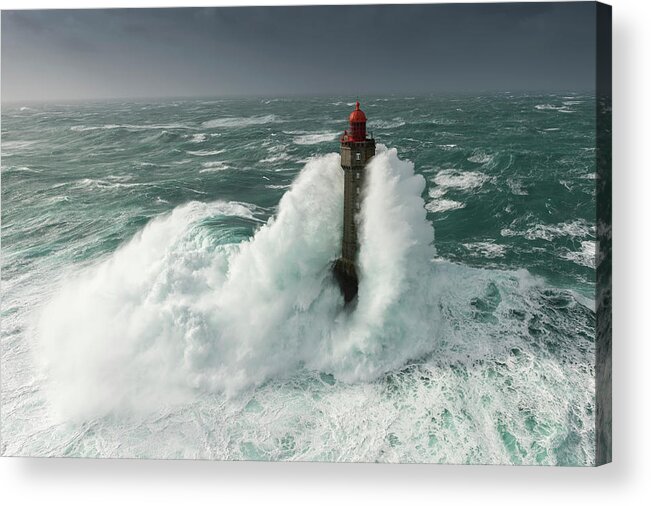This striking canvas-wrapped photo captures a dramatic scene of a lighthouse standing steadfast against the fury of an ocean storm. The lighthouse, a tall cylindrical structure with a dark gray or black facade and topped with a distinctive red cupola, extends upward to about five or six stories. The turbulent sea, a dark green-blue hue with foamy white waves, crashes violently against the base of the lighthouse. On the left side of the image, the waves create misty vapor as they collide with the structure, while on the right side, the foam forms a mesh-like pattern on the water’s surface. Above, the sky is a dynamic canvas of very dark gray clouds that gradually lighten where they meet the horizon, emphasizing the stormy conditions. The scene is vividly captured in this image, which wraps around the right edge of the canvas, making it an immersive and evocative depiction of nature's raw power.